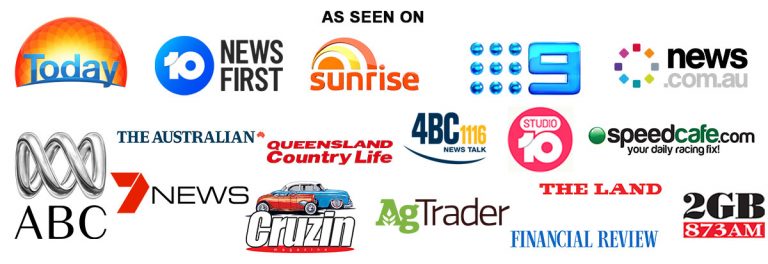This image, sourced from an unspecified origin, features a plain white background with various media logos and captions prominently displayed in black text at the top stating "As Seen On." The logos and corresponding text are arranged as follows:

1. The first icon depicts a rising sun with the text "Today" in blue letters.
2. Adjacent to it, a blue circle with a white number "10" is labeled "News First" in black letters.
3. A semicircular icon labeled "Sunrise" is presented in orange letters.
4. An icon consisting of a 3x3 grid of shiny blue spheres is accompanied by the text "Nine" in blue.
5. A circular icon made up of small, multicolored squares reads "News.com.au."
6. The text "The Australian" appears next, followed by "Queensland Country Life" in red letters.
7. The text "4BC 1116" is labeled as "News Talk" with a black curved line beneath it.
8. A red circle bearing the words "Studio 10" features "Studio" in red letters inside a white text bubble, with the number "10" in white.
9. The words "Speedcafe.com" are labeled as "your daily racing fix," with "Cafe" in green letters and a green dot to the left.
10. A shiny spiral icon carries the text "ABC" beneath it in black letters.
11. The text "7 News" displays a red number "7."
12. The word "Cruzin" is written as "C-R-U-Z-I-N" under an icon of a red car and a blue car.
13. The text "AG Trader" presents "AG" in green.
14. "The Land" is depicted in red letters.
15. "Financial Review" features blue letters.
16. Lastly, the text "2GB 873AM" shows "2GB" in black, with "873AM" in white inside a red rectangle.